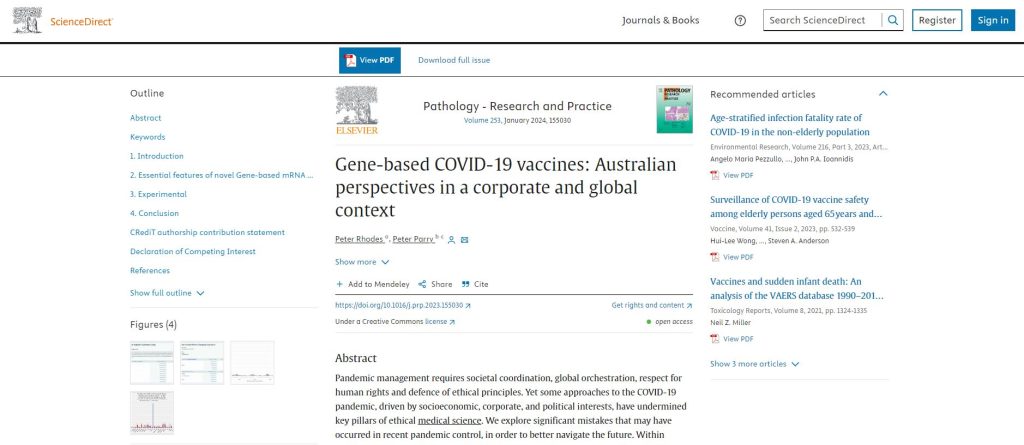Here's a detailed and cleaned-up caption for the image described:

"The image showcases a webpage from Science Direct, featuring a detailed scientific journal article titled 'Gene-Based COVID-19 Vaccines: Australian Perspectives in a Corporate and Global Context,' published in the journal 'Pathology Research and Practice' in January 2024. The page layout includes a navigation pane on the left side, listing sections such as Abstract, Keywords, Introduction, Experimental, and Conclusion, indicating that this is a comprehensive research paper. On the right side of the page, there are recommended articles, including topics like the age-stratified infection fatality rate of COVID-19 in the non-elderly population, surveillance of COVID-19 vaccine safety among elderly persons aged 65 and older, and an analysis of the VAERS database on vaccines and sudden infant death. The top right corner of the webpage features a search bar, a register button, and a sign-in button. The article is published by Elsevier and appears to have two authors."